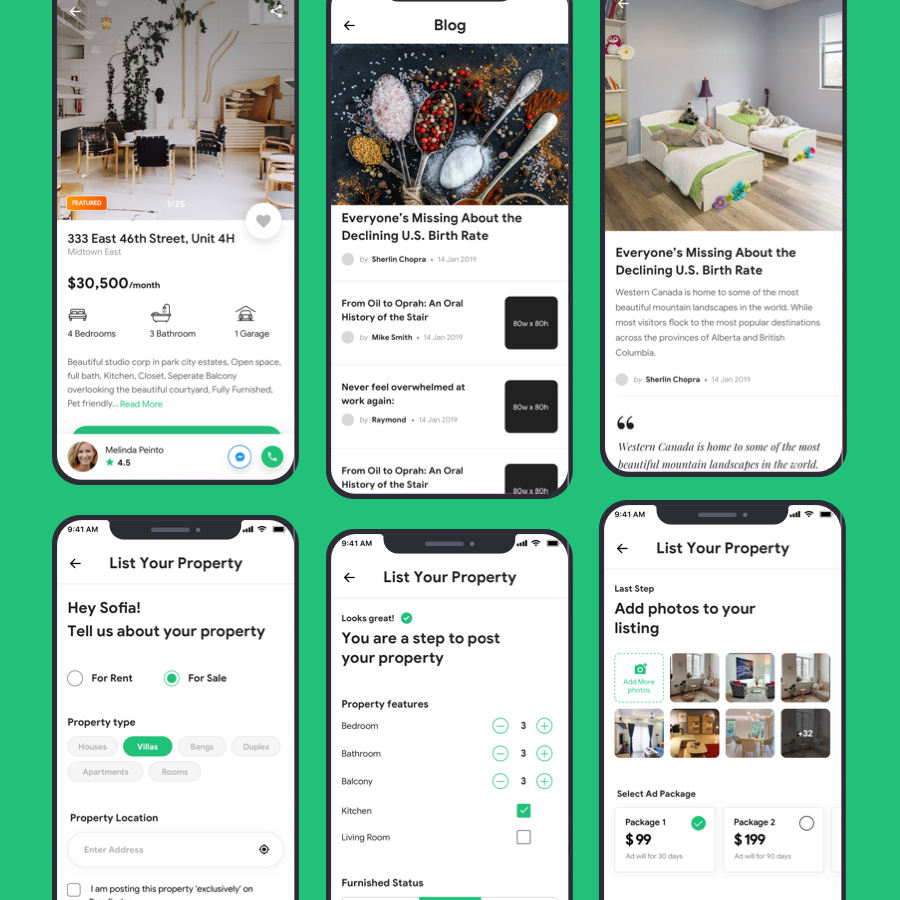The image features a green background with a smartphone displaying six pictures related to property listings and information. Each picture is accompanied by a brief description:

1. **Top Left**:
   - **Property Listing**: Fitch Hat, 33 East 46th Street, Unit 4H, Midtown East
   - **Monthly Rent**: $30,000
   - **Details**: Four bedrooms, three bathrooms, one garage. Includes a beautiful studio, cobbled in park, city estate, open space, full bath, kitchen, closet, separate balcony overlooking the courtyard, fully finished, and pet-friendly.
   - **Design**: Red mode is green with black text.
   - **Seller Profile**: A small profile picture of Melina Painter, rated 4.5 stars. Includes messenger and call buttons which are green.

2. **Center Top**:
   - **Blog Post**: Discusses the declining US pet rate.
   - **Author**: Shirin Chopra
   - **Articles**: "From Oil to Opera: An Oral History of the Stay," "Never Feel Overwhelmed at Work Again."
   
3. **Top Right**:
   - **Article**: "Everyone is Missing About the Declined US Pet Rate"
   - **Background Image**: Two white beds, grey wall, wooden floor with green accents.

4. **Bottom Left**:
   - **Feature**: "List Your Property"
   - **Prompt**: "Hey Sophia, tell us about your property - For Rent or For Sale"
   - **Options**: Property type options including houses, villas, banks, duplexes, apartments, and rooms.
   - **Fields**: Property location.

5. **Bottom Center**:
   - **Step**: "List Your Property"
   - **Message**: "Looks great! You are a step away from posting your property."
   - **Property Features**: Three bedrooms, three bathrooms, three balconies, kitchen checked, living room not checked.

6. **Bottom Right**:
   - **Step**: "Last Step: Add Photos to Your Listing."
   - **Option**: Include images of the property.

7. **Bottom Banner**:
   - **Package Selection**:
     - **Package 1**: $99 (selected)
     - **Package 2**: $199